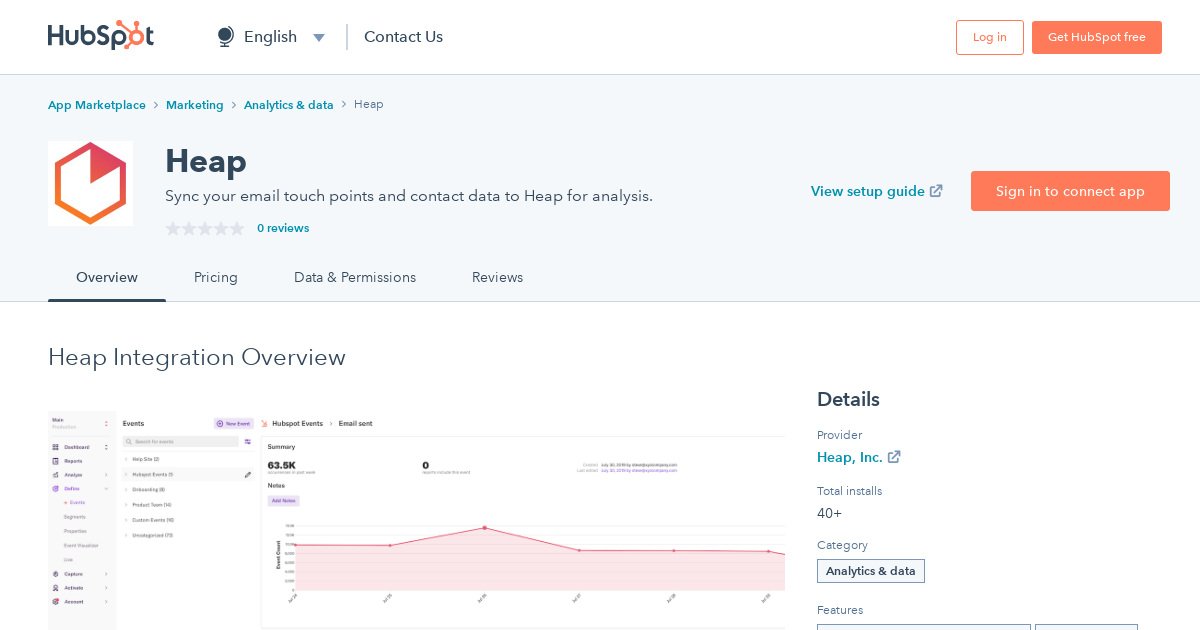This image depicts the HubSpot interface prominently featuring its logo at the top. The "HubSpot" text is spelled out, with the 'O' designed in orange and including three lines extending outward—one upward, one to the left, and two additional lines to the left. The top-most line is longer and adorned with small circles.

To the right of the logo, there is a navigation bar. On the left, it starts with a globe icon labeled "English" with a downward-pointing arrow, followed by a "Contact Us" link. On the far right, there are two buttons: the "Login" button with orange lettering on a white background, and next to it, an "Get HubSpot Free" button showcasing white lettering on an orange background.

Below this navigation bar is a long, grayish background bar containing several blue text links including "Marketplace," "Marketing," "Analytics," and "Data." The word "HEAP" is displayed in a grayish color. Beneath this, there’s an icon shaped like an octagon or hexagon with an orange or reddish triangle inside it. Next to this icon, "HEAP" is written in black letters followed by the text: "Sync your email, touch points, and contact data to HEAP for analysis." Adjacent to this text is a blue link reading "View Setup Guide," and an orange button with white lettering stating "Sign in to connect app."

Further down, below the HEAP integration information, there are five unhighlighted stars accompanied by the text "0 reviews." Underneath, there are four tabs labeled "Overview," "Pricing," "Data and Permissions," and "Reviews," all in black lettering.

Lastly, the section titled "HEAP Integration Overview" is followed by a red grid providing a summary of details and notes. This section is further broken down with detailed sub-sections labeled "Details" in black lettering, including information about the provider: "HEAP Inc," total installs: "40+," category: "Analytics and Data," and a list of features.